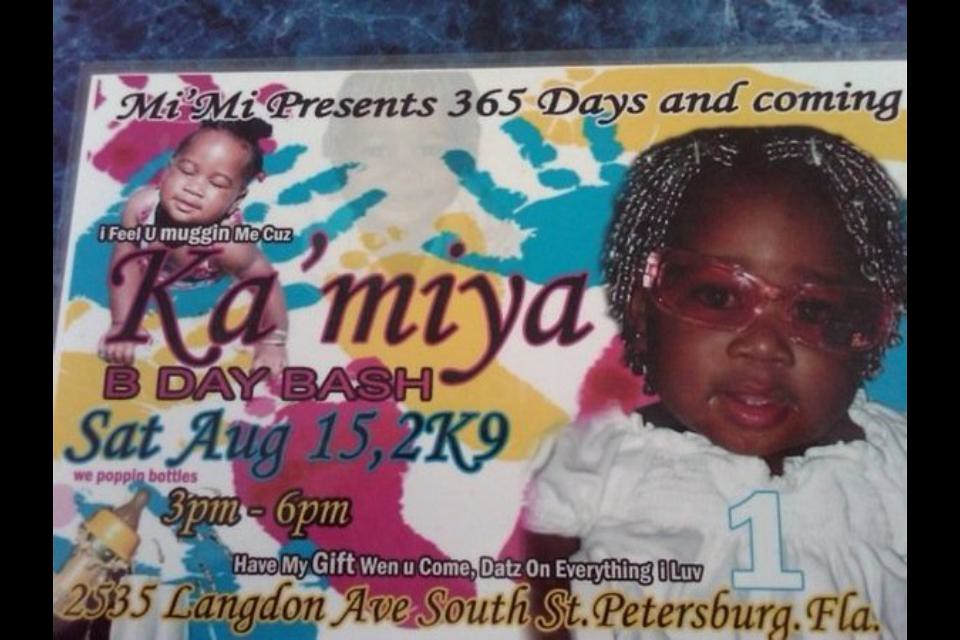In this vibrant birthday invitation, a little girl named Kamaya is celebrated. The background is scattered with colorful handprints and footprints in yellow, red, and teal. At the top of the invitation, in a somewhat cursive and playful font, it reads, "Mimi Presents: 365 Days and Counting." On the left, a smaller image of Kamaya shows her crawling with eyes closed, while on the right, a larger photo captures her wearing pink glasses and a white frilly top, with a bold number "1" indicating her milestone year. The invitation details Kamaya's Birthday Bash on Saturday, August 15, 2009, from 3 PM to 6 PM at 2535 Langdon Avenue, South St. Petersburg, Florida. The text humorously adds, "We poppin' bottles," inviting guests to bring gifts in a playful tone.